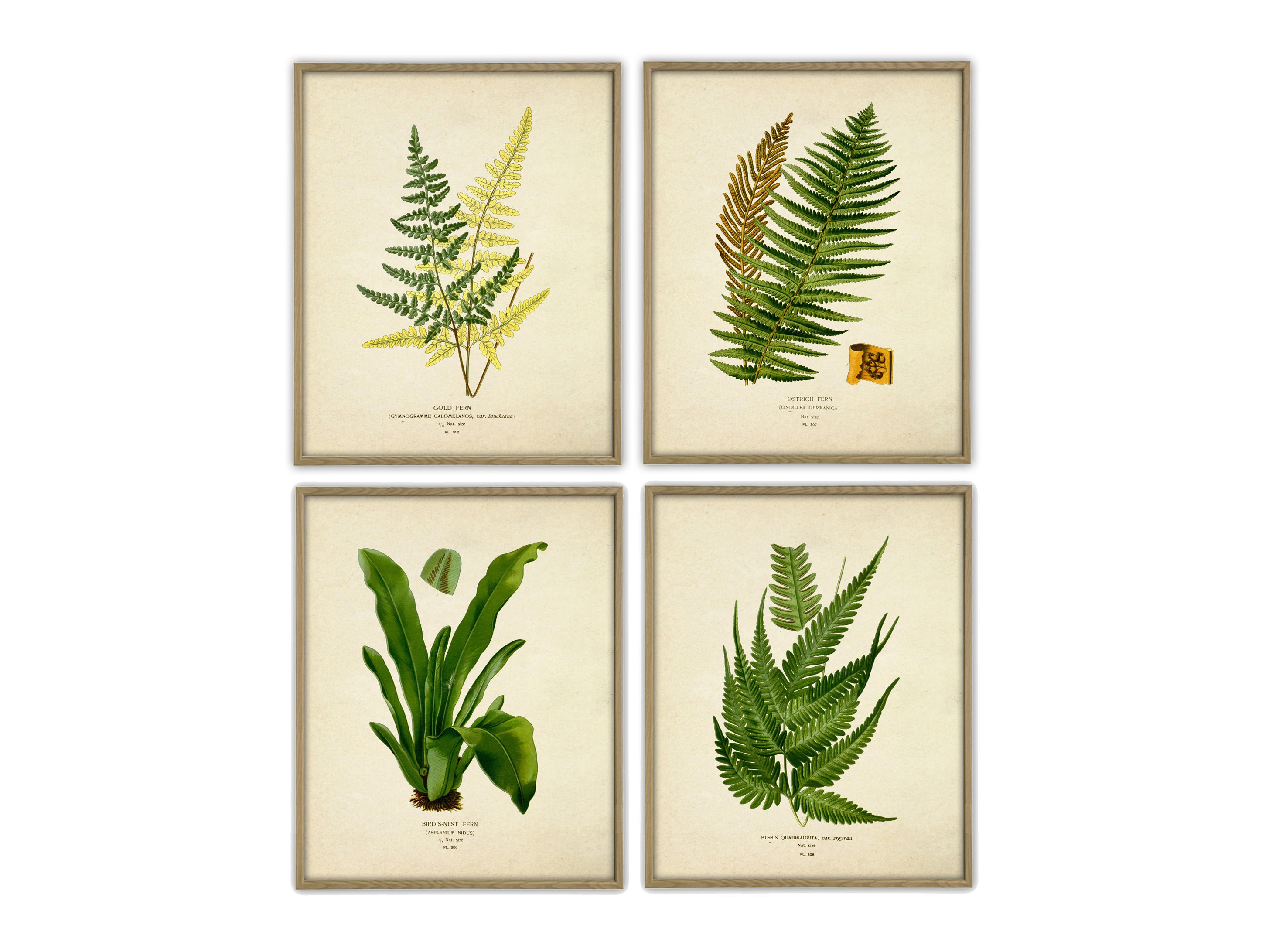The image consists of four framed botanical illustrations arranged in a 2x2 grid on a pure white background. Each frame is made from a modern grayish wood and contains a botanical drawing with a parchment-like, yellowish-cream background. Though the text beneath each plant is too small to read, the detailed illustrations appear realistic, reminiscent of those found in a botanical garden guide. 

In the top row, the first frame features a fern with light green fronds, while the second frame also contains a fern but with thicker, more substantial fronds, one green and one browner in tone. The bottom row has another fern in the left frame, characterized by vivid green leaves extending in various directions. The final frame on the bottom right showcases a different type of plant, possibly not a fern, with taller, flatter green leaves that bend gracefully at the tips. Notably, the top right image carries a distinct orange scroll logo with illegible black text, adding a unique element to the composition. Each image holds intricate details, contributing to the overall impression of meticulously crafted botanical art.